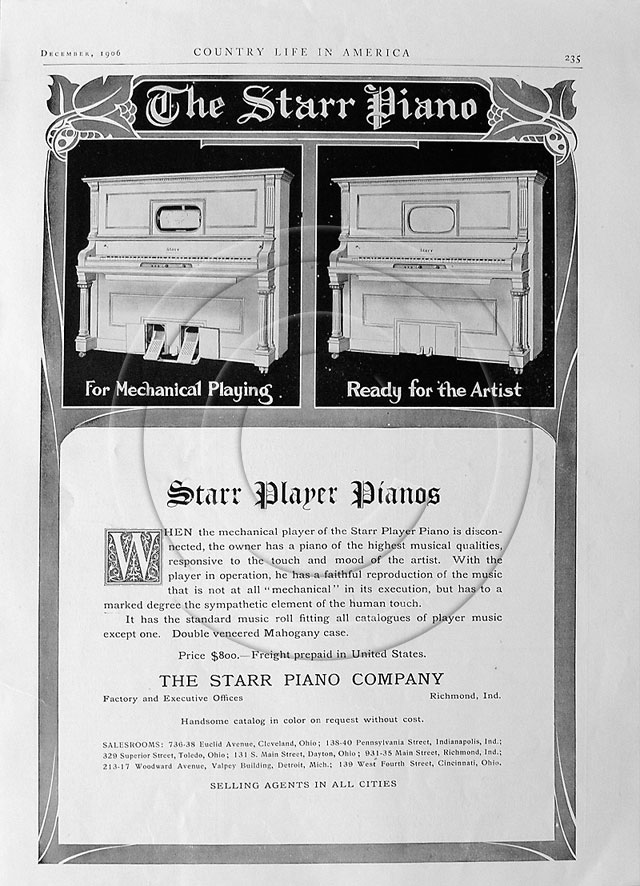This image is an archived advertisement from December 1986, likely extracted from page 235 of Country Life in America. The advertisement is set on a white or light gray background, enclosed within an ornate gray border. At the top, "Country Life in America" is printed in black, and below it, "The Star Piano" is prominently displayed in white font against a black background, flanked by intricate leaf designs.

Two images of the Star Piano are featured: the left image shows a larger piano with prominently exposed foot pedals, labeled "For Mechanical Playing," while the right image is labeled "Ready for the Artist," depicting a similar piano with less visible foot pedals. Below these images is a detailed description set against a white background, titled "Star Player Pianos." It states: "When the mechanical player of the Star Piano is disconnected, the owner has a piano of the highest musical quality, responsive to the touch and mood of the artist. With the player in operation, he has a faithful reproduction of the music that is not at all mechanical in its execution, but has to it a marked degree the sympathetic element of the human touch. It has the standard music roll, fitting all catalogs of player music except one, double-veneered mahogany case. Price, $800. Freight prepaid in the United States." 

Further down, the text notes: "The Star Piano Company. Factory and executive offices, Richmond, Indiana. Handsome catalog in color on request without (unreadable text)." The bottom of the advertisement includes the phrase "Selling agents in all cities" and features a transparent logo resembling a copyright "C" shape.